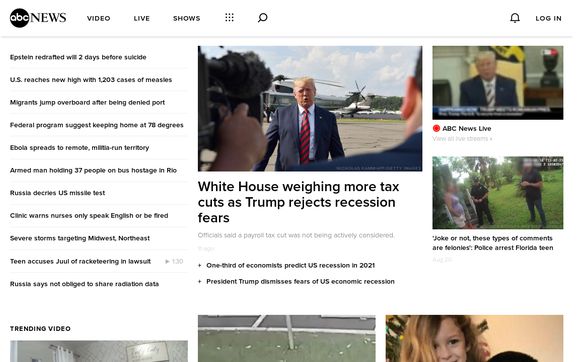The image showcases a detailed snapshot of the ABC News webpage. In the upper left corner, the ABC News logo is prominently displayed, accompanied by navigation options that include "Video," "Live," and "Shows." Down the left column, a series of headlines capture significant events and updates: 

1. "Epstein Redrafted Will Two Days Before Suicide"
2. "U.S. Reaches New High With 1,203 Cases of Measles"
3. "Federal Program Suggests Keeping Home at 78 Degrees"
4. "Russia Decries U.S. Missile Test"
5. "Clinic Warns: Nurses Only Speak English or Be Fired"
6. "Severe Storms Targeting Midwest Northeast"
7. "Teen Accuses Jewel of Racketeering in Lawsuit"

Centrally positioned on the page, there is a picture of President Donald Trump near a helicopter, engaged with reporters. The accompanying headline reads: "White House Weighing More Tax Cuts as Trump Rejects Recession Fears." Below this, additional text notes: "One Third of Economists Predict U.S. Recession in 2021. President Trump Dismisses Fears of U.S. Economic Recession."

On the far right, there's another image of Donald Trump, garbed in a suit, taken during his presidency in the White House. This section is marked by a "Live" indicator featuring a red dot, labeled "ABC News Live." 

Beneath this, an outdoor photo captures a scene with at least one police officer and a civilian to the left of the officer. This image is captioned: "Joke or Not, These Types of Comments Are Felonies. Police Arrest Florida Teen."

The compilation of images and headlines offers a comprehensive glimpse into a range of current national and international news stories, economic predictions, and policy discussions.